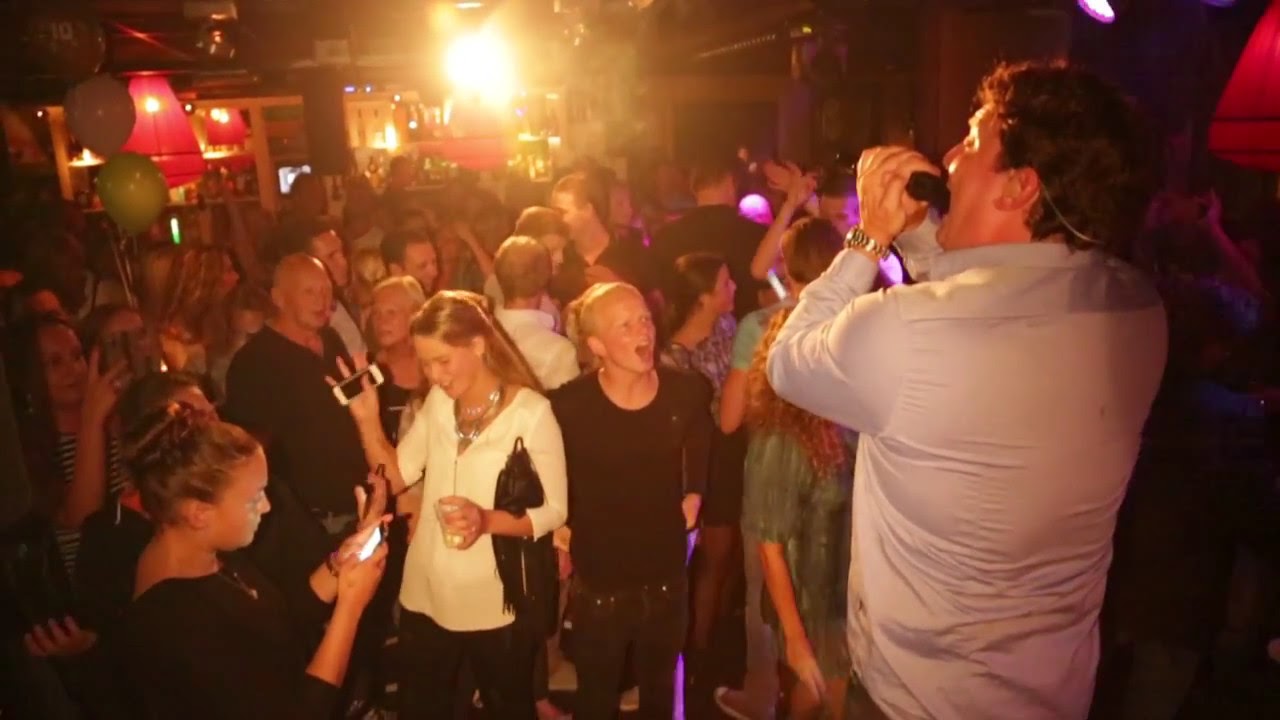The image captures a vibrant birthday celebration at a club, teeming with young people reveling in the energetic atmosphere. Multicolored balloons—green, pink, and purple—adorn the background, contributing to the festive vibe. A charismatic man at the forefront, wearing a light blue collared shirt and a silver wristwatch on his left wrist, holds a microphone to his mouth, seemingly rallying the crowd with spirited shouts or possibly singing. His brown hair and visible enthusiasm add to the dynamic scene. The club is bathed in light, with red lamps hanging from the ceiling, and several attendees are capturing the moment on their phones, indicating their engagement with the performance. To the side, a bar area with a glimpse of bottles can be spotted. In front of the performer, a woman in a white top, adorned with silver jewelry, holding a glass and her phone, stands alongside other enthusiastic onlookers, some of whom are joining in with the singing. The lively backdrop of lights and a sea of joyous faces encapsulates the essence of a jubilant club birthday party.